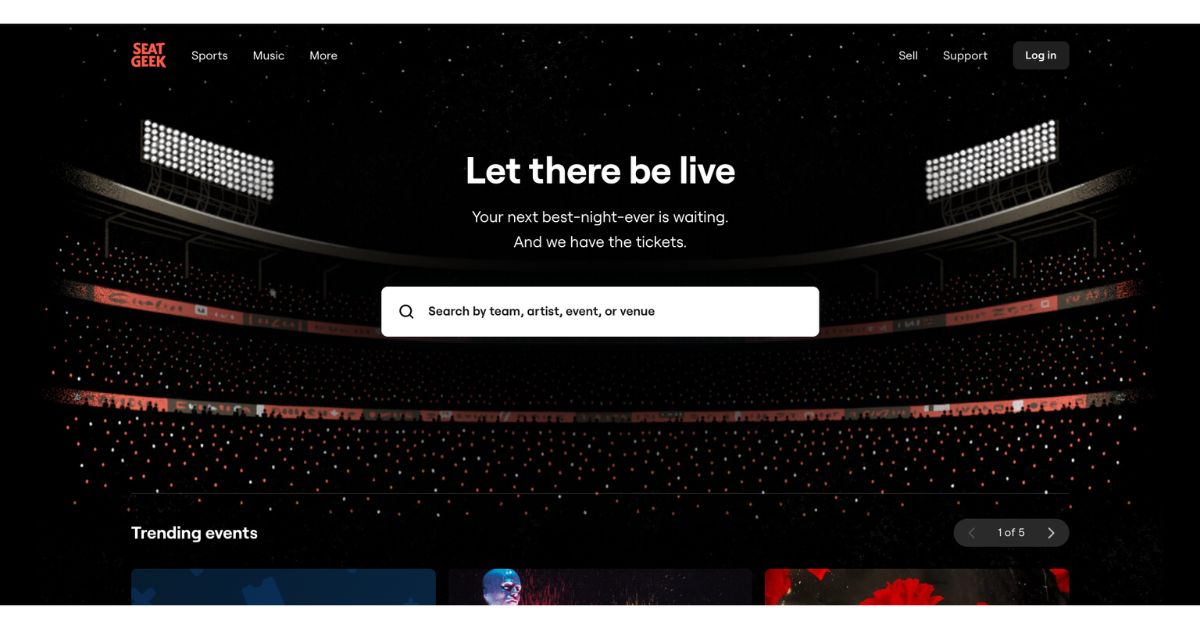The image appears to be a screenshot from the SeatGeek website, featuring a sleek design with a black background reminiscent of a sports arena. In the upper right corner, the SeatGeek logo is prominently displayed in red, followed by the categories "Sports Music More," "Cell Support," and a "Login" button. Centered in the middle of the screen is the bold, white text "Let There Be Live," accompanied by the subtitle "Your Next Best Night Ever is Waiting and we have the tickets." Below this, a large search bar invites users to "Search by Team, Artist, Event, or Venue."

The background design subtly depicts an arena filled with small white and red dots representing spectators, and lights positioned at the top left and right corners illuminate the scene. In the bottom left corner, the phrase "Trending Events" is visible in white text. Meanwhile, the bottom right corner features an oval-shaped indicator "1 of 5" with a right-pointing triangle, suggesting a carousel of images. Three partially visible images at the bottom of the screen include a gray, indistinct picture, an Android-type face of a bald man with a silver head, and a third image depicting a black background with what appears to be a red flower.